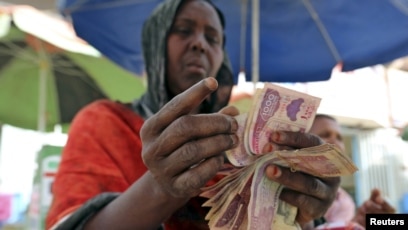The photograph captures a close-up of a black woman with darker skin, intently counting a large stack of colorful foreign currency bills, one of which prominently features the denomination "10,000" and is light purple. She wears a thin, dark brownish material draped over her head like a hijab, though it does not cover her entirely, along with a reddish-orange outfit. The scene is set under the protection of umbrellas, with a blue umbrella shielding her directly and a green and off-white alternating umbrella visible behind her, indicating she might be in a street market. The presence of the "Reuters" watermark in the bottom right corner suggests this image was captured by a Reuters photographer. A person’s face is partially visible in the background, adding to the bustling market atmosphere implied by the umbrellas and the casual environment.